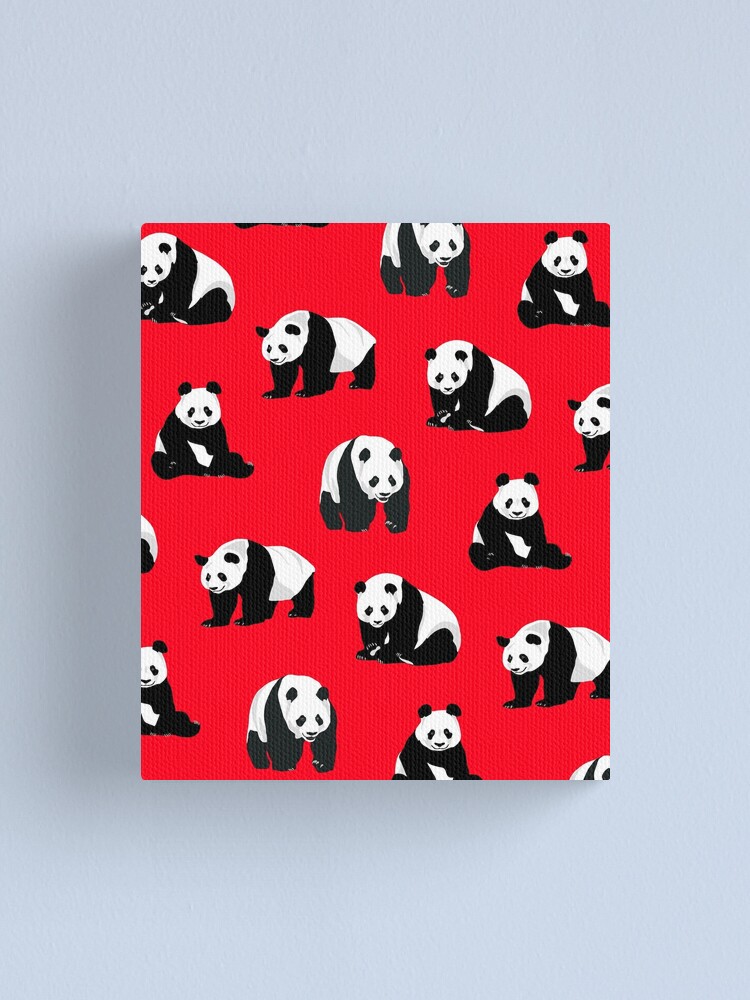This image is a photographic graphic depicting an array of approximately 15 black and white panda bears in various positions. Set against a light-colored, possibly blue or gray, background, the focal point is a bright, orangey-red square print adorned with these pandas. The red square is vivid and prominently contrasts with the overall scene, which may give the impression of a box, wrapping paper, or a swatch of material. 

The pandas are drawn in a sketch-like style and are seen in diverse postures: sitting, standing on all four legs, standing upright, and leaning forward while seated. Each panda is oriented differently, with some facing straight ahead and others turning left or right. Notably, some pandas are partially obscured, especially those at the edges of the red square, contributing to the visual complexity of the design. There is no text on the image, enhancing the striking visual appeal of the black, white, and red composition.